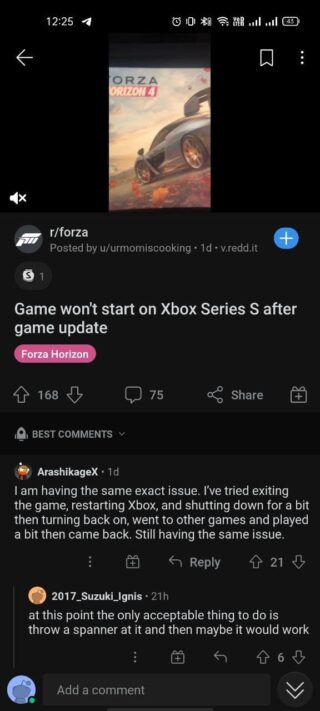In this detailed screenshot of a mobile phone, captured at 12:25 PM, various interface elements are displayed. The status bar at the top shows typical phone indicators such as signal strength, battery life, and notification icons. Below the status bar, there's a navigation arrow pointing left, a bookmark icon, and a vertical ellipsis (three dots), which likely represents a menu option.

The core content of the screenshot is a post on Reddit, specifically from the subreddit r/forza, which focuses on the popular racing game Forza. The subreddit has a small image displaying the title "Forza Horizon 4" with a picture of a car, indicating the game being discussed.

The post is authored by the user "u/(u momascooking)," referencing their username with a playful twist. The post’s title reads, "Game won't start on Xbox Series S after game update," hinting at a technical issue being faced by the user. Accompanying this, the post is categorized under "Forza Horizon," highlighted in a pink tag.

Engagement metrics show an upvote count of 168, with no downvotes, and the post has attracted 75 comments. Interaction options include buttons for upvoting, downvoting, sharing, and gifting awards, indicated by a present icon.

The section under the post features the best comment, written by "Arashish Kaji X" a day ago. At the very bottom of the screen, there's an option to add a comment, encouraging further discussion.